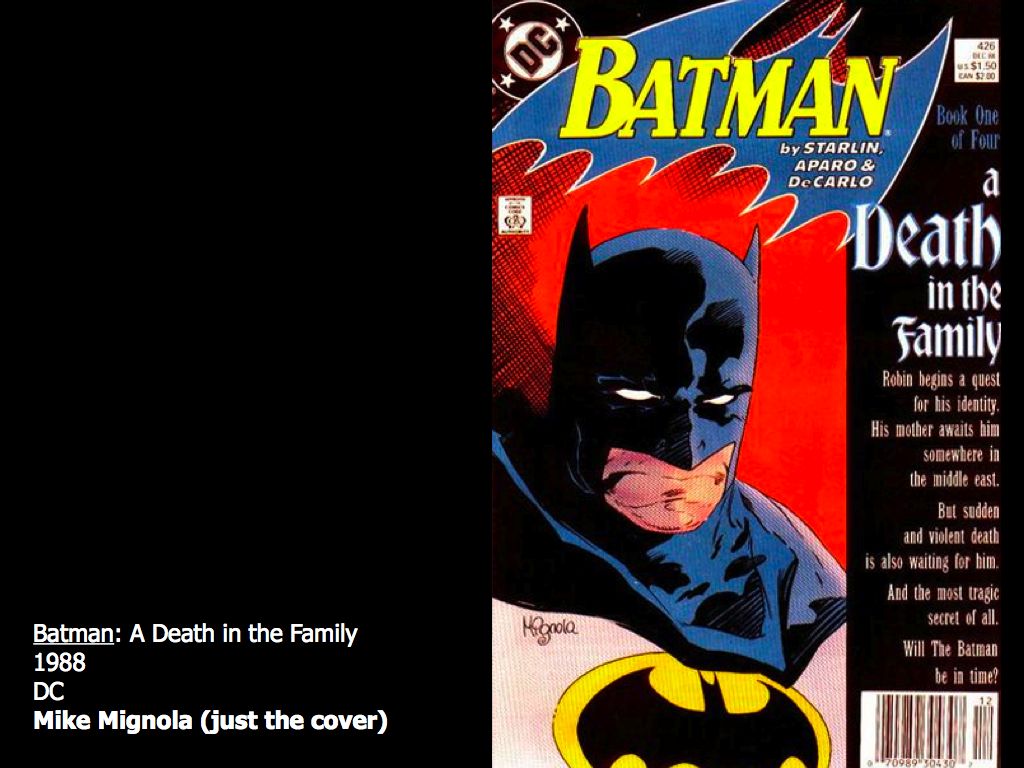The image showcases the front and back covers of a Batman comic book laid flat. The left half, which is entirely black except for white text at the bottom, reads: "Batman, A Death in the Family, 1988, DC, Mike Mignola (just the cover)." The right half features the striking cover art. At the top, a circular DC logo is present. Below it, "Batman" is prominently displayed in bold yellow font over the classic Bat-Signal, depicted as a blue bat shape outlined in white. The cover illustration features Batman with his ominous, beady eyes. To the right, a white font against a black banner reads: "A Death in the Family." Additional text on the right mentions Robin's quest for identity and the perilous journey awaiting him in the Middle East, hinting at a tragic unfolding. A barcode is situated in the lower right corner of the cover. The creative team behind this iconic comic includes Starlin, Aparo, and DiCarlo.